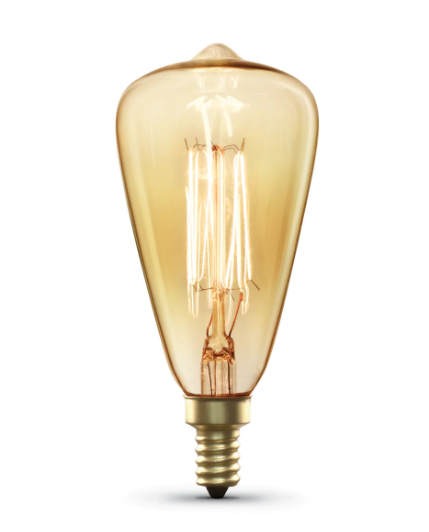This is a photograph of an unusual vintage-style light bulb with a distinctly modern twist. The core center of the bulb is small and twists in, while the internal antique filament structure gives it a retro aesthetic. The shape of the bulb resembles an elongated upside-down egg, diverging from traditional bulb shapes. Illuminated with a golden, amber hue, it features a goldish, tan, and beige coloring, reminiscent of a Caucasian nude palette. The bulb is designed for smaller sockets, approximately the size of a lead pencil, and is commonly used in fixtures like chandeliers that require multiple bulbs. While it emulates an old-fashioned, incandescent look, the bulb incorporates modern lighting technology. The bottom features a gold coil resting on a semi-spherical base, casting a shadow on a white surface below, which dominates the composition of the image.